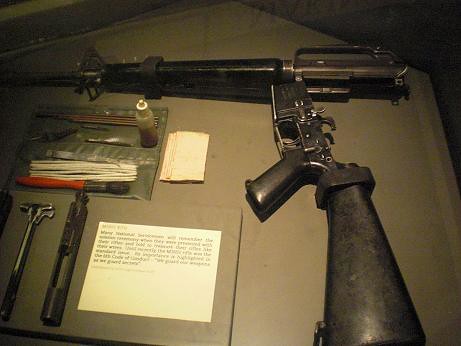In a dimly lit room, a glass case houses a meticulously arranged museum display of a vintage rifle. The firearm, which appears to be an antique assault rifle or shotgun, is presented in two separate parts: the black barrel and the associated trigger mechanism. Accompanying the rifle are various maintenance tools, including what seems like a hammer for adjustments on the bottom left, and several bottles presumably for lubrication and cleaning purposes. There's also an additional chamber for ammunition. A small white sheet of paper with tiny, unreadable text provides information about the exhibit. The overall ambiance is quite dark, with only a light above the display illuminating the intricate details of the rifle and its accessories.